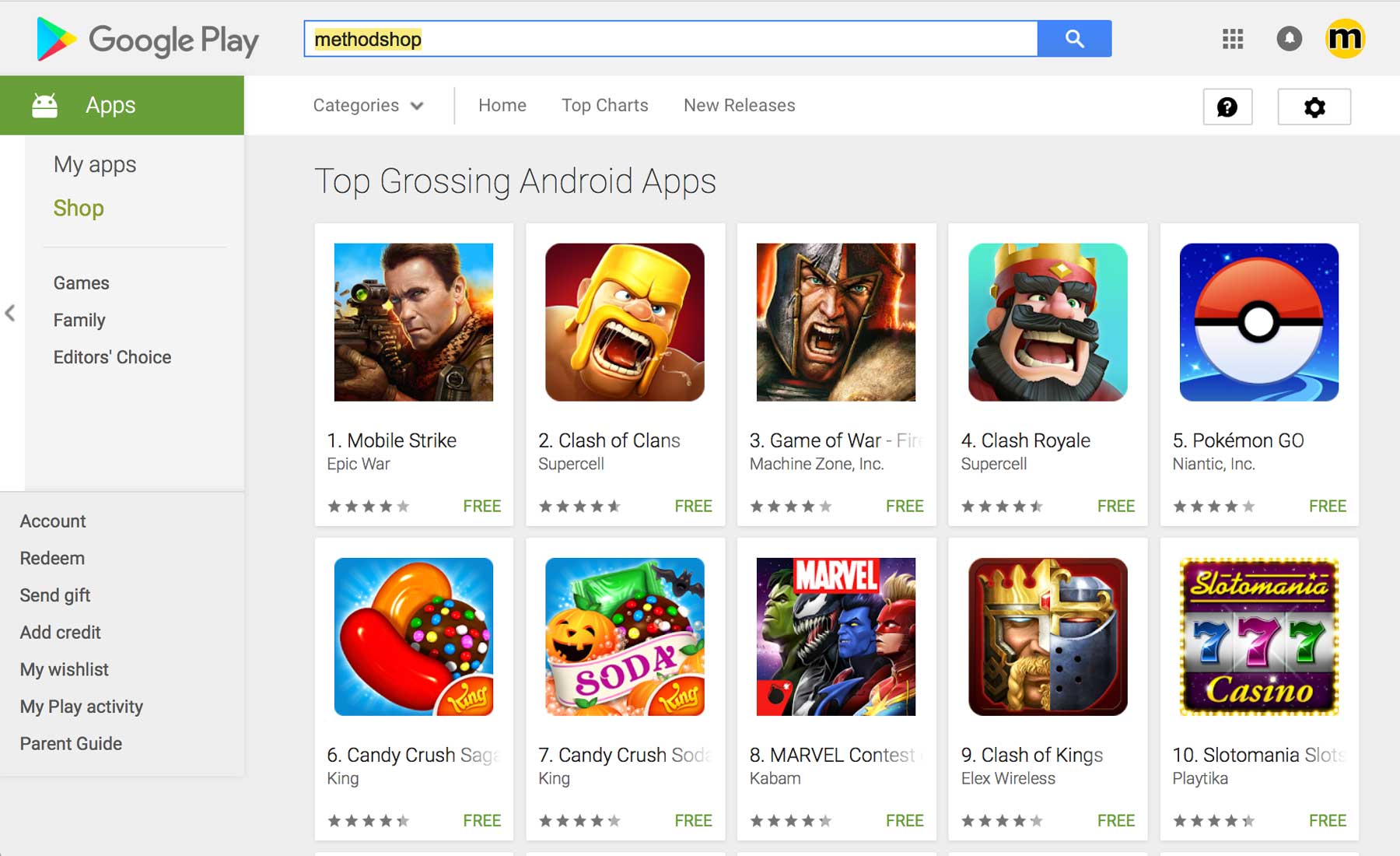The screenshot captures a horizontal image of a web page from the Google Play store. In the upper left-hand corner, the recognizable Google Play icon and text "Google Play" are prominently displayed. To its right sits a search bar with a light yellow background, where the term "Method Shop" has been entered. Adjacent to the search bar, three icons are neatly aligned, forming part of the top header bar.

The row beneath the search bar features navigation categories, including "Categories," "Home," "Top Charts," and "New Releases," with two additional buttons positioned towards the right of this header section. A vertical navigation bar on the left-hand side indicates that the "Apps" section is currently highlighted. Other categories listed in this sidebar include "My Apps," "Shop," "Games," "Family," and "Editor's Choice." Towards the bottom of the sidebar, additional options such as "Account," "Redeem," "Send Gift," "Add Credit," "My Wishlist," "My Play Activity," and "Parent Guide" are labeled.

Dominating the main portion of the page is the “Top Grossing Android Apps” section, showcasing 10 small game icons arranged sequentially from 1 to 10. The highlighted games in this roster are: "Mobile Strike," "Clash of Clans," "Game of War," "Clash Royale," "Pokemon Go," "Candy Crush," "Candy Crush Soda King," "Marvel Contest," "Clash of Kings," and "Slotomania Slots."